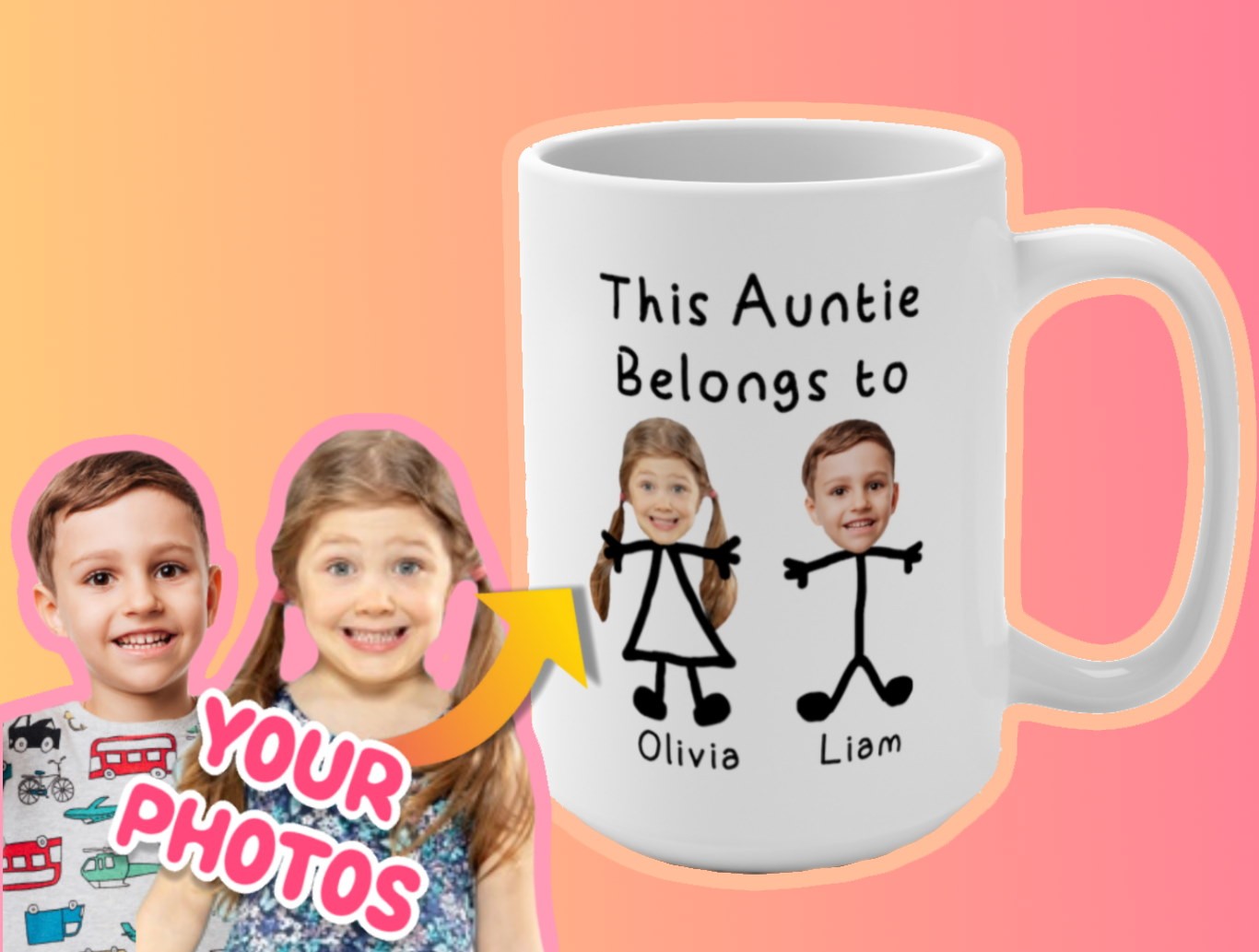This advertisement showcases a customizable coffee mug set against a gradient background transitioning from orange to pink. In the bottom left corner, it features two young children—a boy with short hair and a white shirt adorned with red cartoon buses and planes, and a girl with pigtails wearing a turquoise summer dress with white flowers. The children are making goofy, smiling faces. 

An arrow in yellow with the text "Your Photos" in pink points towards the white coffee mug. The mug is designed to allow personal photos to be superimposed onto stick figures drawn in black. The mug reads, "This auntie belongs to Olivia and Liam" in black text, with the children's faces depicted on the stick figures. One stick figure is standing plainly, while the other is accompanied by grass. The two kids in the corner also have a subtle pink outline around them, enhancing the cohesive design of the entire advertisement.